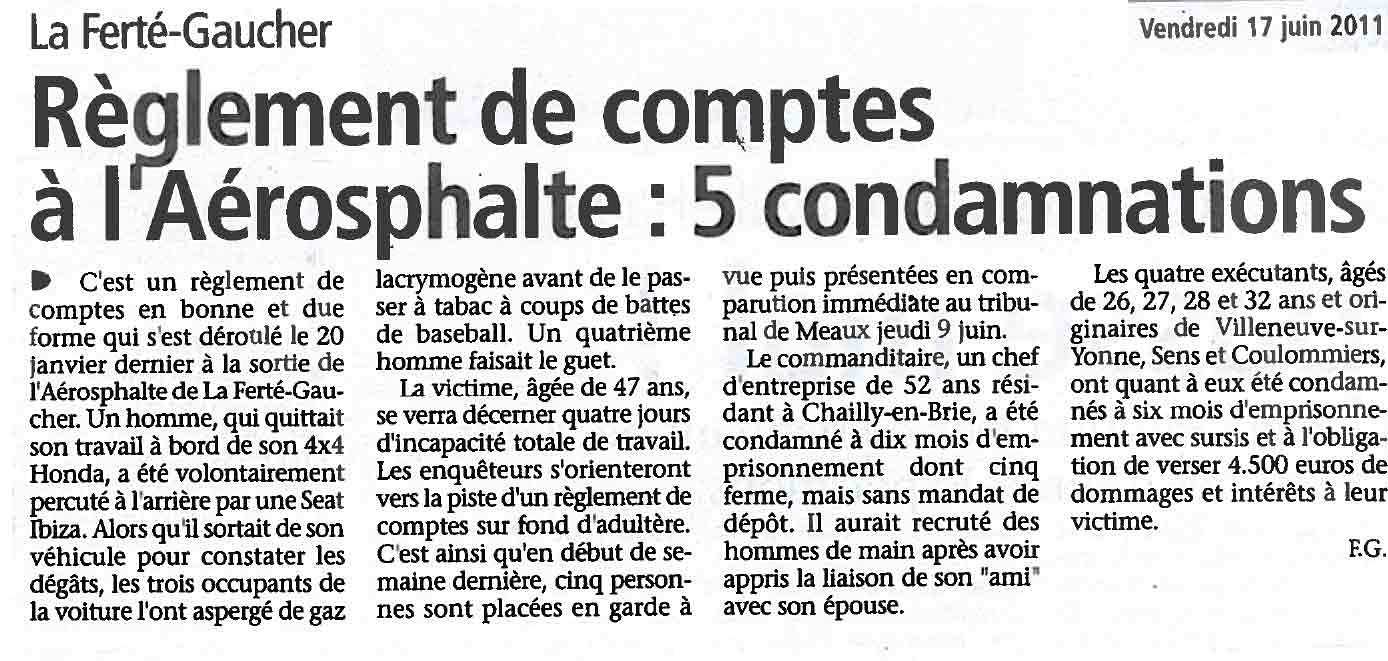The image depicts a black and white excerpt from a French newspaper article dated Vendredi 17 Juin 2011 (Friday, June 17, 2011). The headline reads "Règlement de Compte à l'Asphalte, Cinq Comptes d'Annation." The article, likely about some regulatory matter, is composed of four paragraphs arranged in columns. The byline, located in the top left corner, corresponds with the initials E.G. found at the end of the text, possibly indicating the author's name or the newspaper title, La Ferté Gaucher. The text is clear but slightly blurred, suggesting the image might be a photograph, photocopy, or printout.